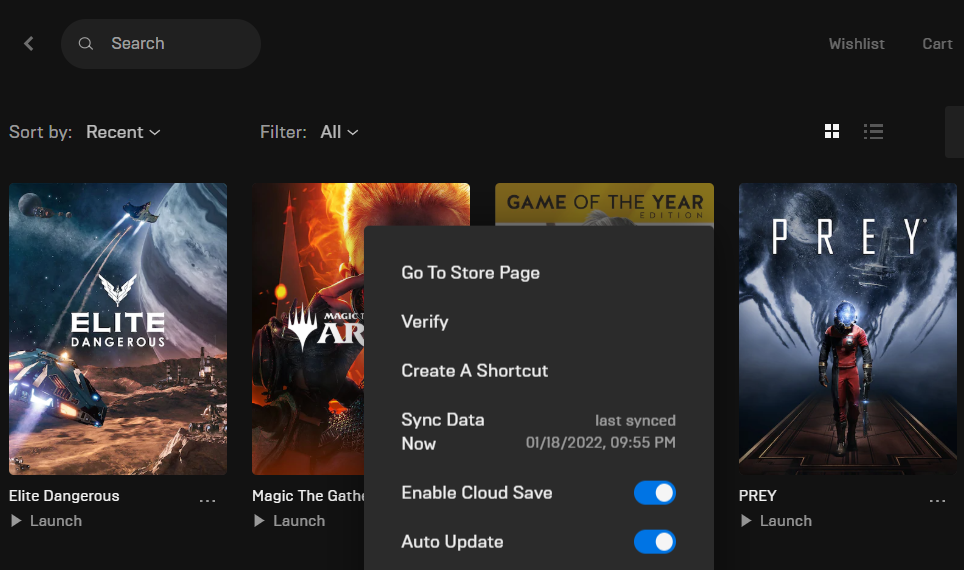A detailed screen capture from a webpage featuring a selection of video games. The background displays a row of game thumbnails, each representing different titles. On the left, the game "Elite Dangerous" is shown, with an image of spaceships flying through space and a "Launch" button beneath it. To the right, another game titled "Prey" features a man in a spacesuit facing an alien, also accompanied by a "Launch" button.

In the center of the screen, there is an overlay with a black square, displaying options such as "Go to Store Page," "Verify," and "Create a Shortcut." Further down, it provides synchronization details, stating "Last Synced: 01/18/2022 at 9:55 PM." Below this, there are settings for "Enabled Cloud Save" and "Auto-update," each with a blue oval toggle button to their right. This interface suggests users can store game data to the cloud and ensure games are updated automatically, facilitating gameplay at a later time.